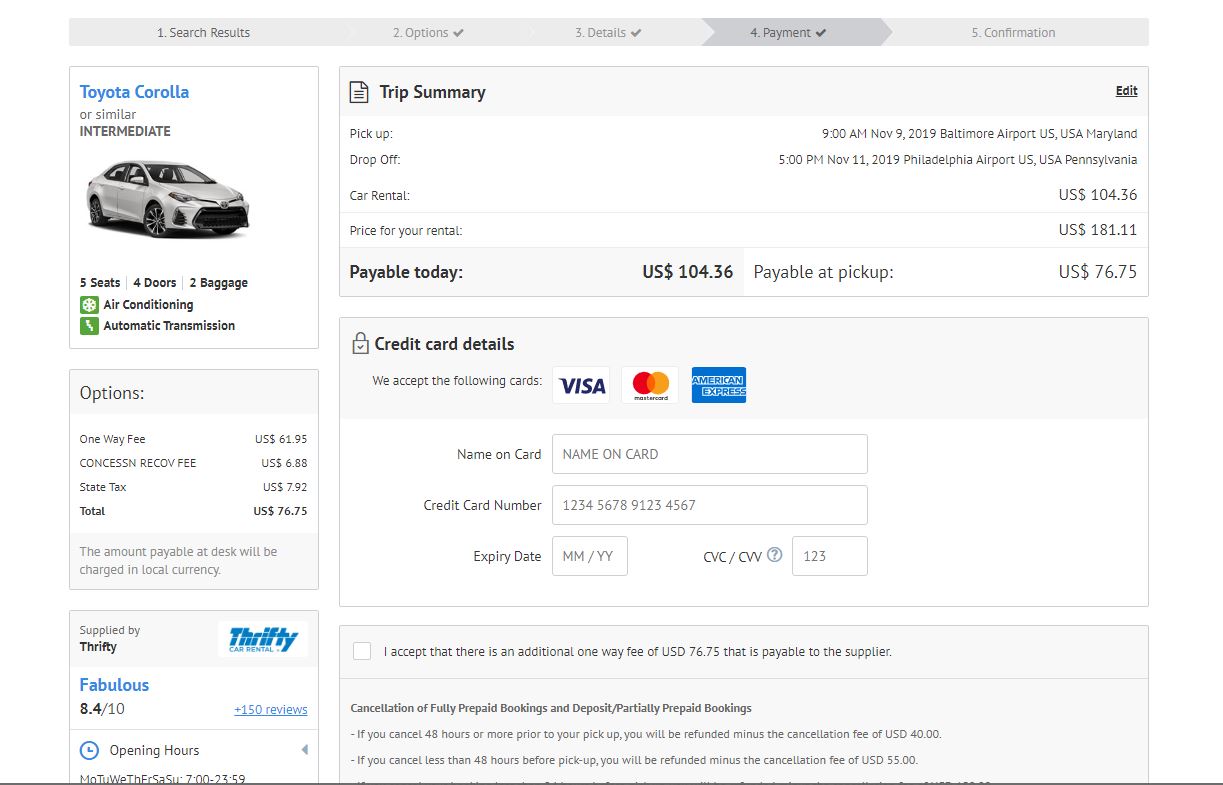The image displays a website interface specializing in vehicle rentals, prominently featuring a Toyota Corolla. The layout is organized into a sequential navigation bar at the top, indicating different stages of the booking process, all of which have been checked off except for the final step. 

1. At the top-left, marked with the number "1," is the "Search Results" tab.
2. To its right, the number "2" signifies the "Options" tab, accompanied by a check mark. 
3. Continuing horizontally across the top-middle section, the number "3" highlights the "Details" tab, also checked.
4. Further right, the "Payment" tab is indicated by the number "4." This tab stands out with a slightly darker gray background, also marked with a check mark.
5. The final stage, "Confirmation," is marked as number "5" and positioned at the top-right corner.

On the left side, near the top, inside a box with blue text, is the label "Toyota Corolla." Below this, an image of a Toyota Corolla vehicle in a grayish-white hue is displayed. The description beneath the image identifies it as having three seats, four doors, and space for two bags, featuring air conditioning and an automatic transmission.

Centrally positioned in the middle section of the image is the "Trip Summary," detailing costs. It indicates an immediate payment amounting to $104.36, with an additional listing to the right showing a U.S. dollar amount of $76.75.